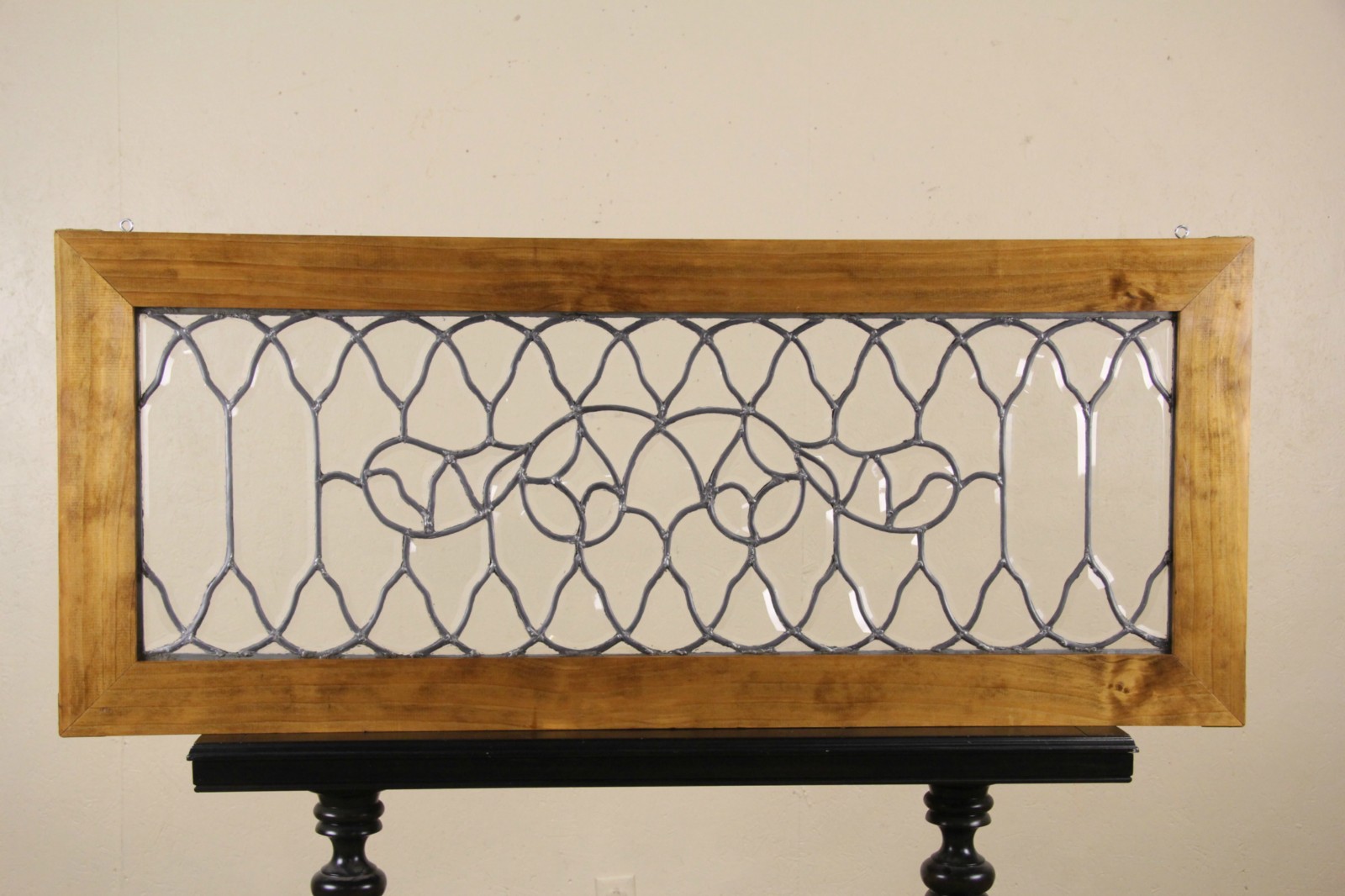The image showcases a rectangular, orangish-brown wooden frame set against a beige, light-pinkish background. The frame features a randomly woven, intricate metal design in the center, resembling a winding snake. Inside the frame, there appears to be clear glass, evidenced by slight reflections. The frame is positioned on a small black wooden bench, which is not as long as the frame itself. The bench has two ornate legs, reminiscent of pawn chess pieces, though their bottoms are cut off in the image. The frame also has two small eye hooks at the top, suggesting it could be suspended, possibly by invisible fishing line, as one might with a transom window. The detailed craftsmanship and design evoke a Victorian aesthetic, making it appear as a beautiful decorative piece suitable for such a style.